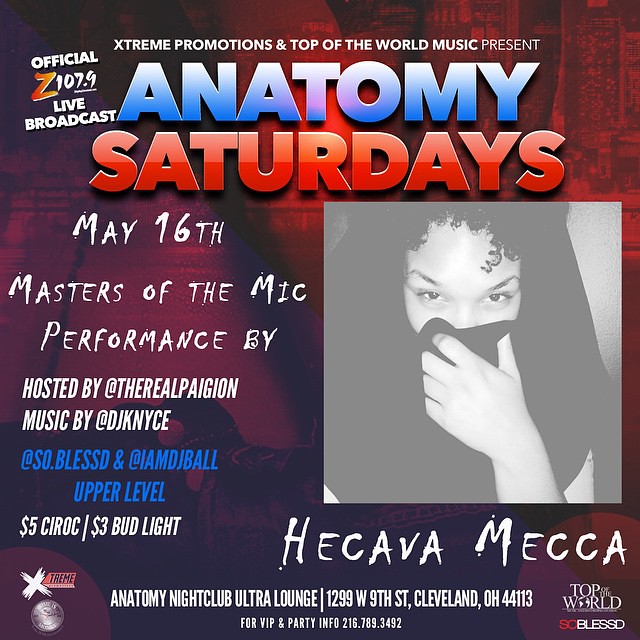This image is a detailed promotional poster for an event at Anatomy Nightclub and Ultra Lounge, primarily showcasing a Black and white photo of an African descent woman centered to the right side. She has curly hair falling over her forehead and holds a scarf across the lower half of her face, staring directly at the camera. The background transitions from red at the upper right to a purple-plum hue toward the lower left, adding a dramatic effect. 

At the top, the poster reads "X-treme Promotions and Top of the World Music Present," in white print, followed by "Official Z107.9 Live Broadcast" where the 'Z' is highlighted in red and orange. Below this, in bold blue lettering, it states "Anatomy" and in bold red "Saturdays." The details continue with the date "May 16th" and the event "Masters of the Mic Performance by." The host is mentioned as "The Real Pagean," with music by "DJ K Nice" and additional performances by "@SOSO.Blessed and @IMMDJBALL, Upper Level Concert."

Further details include drink specials "$5 C-Rock/$3 Bud Light" and the location "1299 West 9th Street, Cleveland, Ohio 44113." For VIP and party information, it lists the phone number "216-789-3492." The lower sections also feature the logos for Xtreme, Top of the World, and So Blessed. The color palette of the poster consists of black, white, blue, red, orange, gray, and maroon, creating a vibrant and eye-catching announcement for the upcoming event.